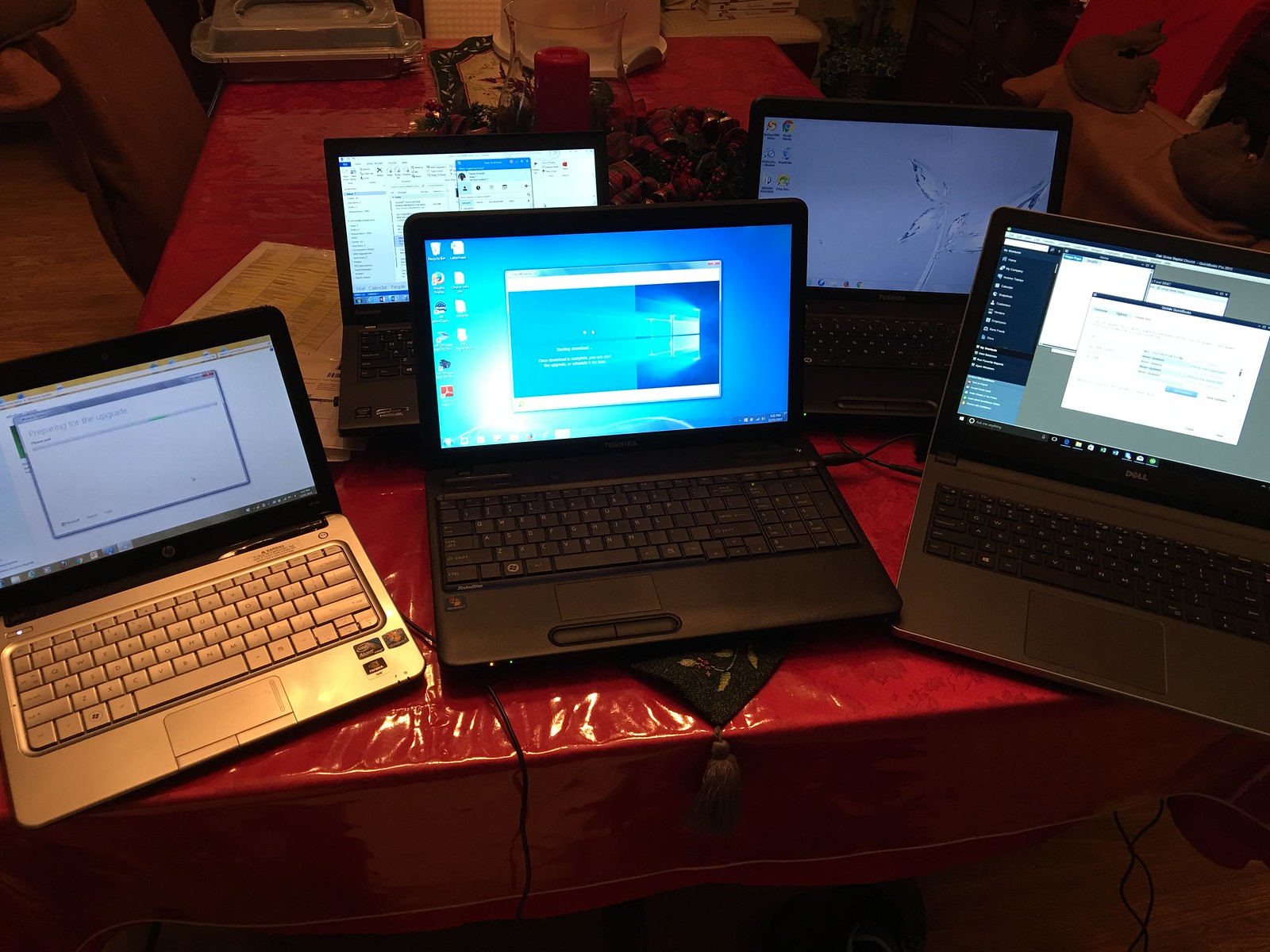The image depicts five open laptops arranged on a long table covered with a shiny red tablecloth. Each laptop is turned on, displaying a variety of screens and programs. Four laptops have black keyboards, while the fifth one, positioned on the left, features a silver keyboard. The center laptop shows a blue background with several icons and an open window, the leftmost laptop seems to be loading, and the laptop to the right displays three open windows. Toward the back of the table, there's one laptop with windows open, and another with a plain silver background. The table is adorned with a centerpiece consisting of a red candle surrounded by small rocks, and a small black cloth is placed under one of the central laptops. In the background, chairs are faintly visible.